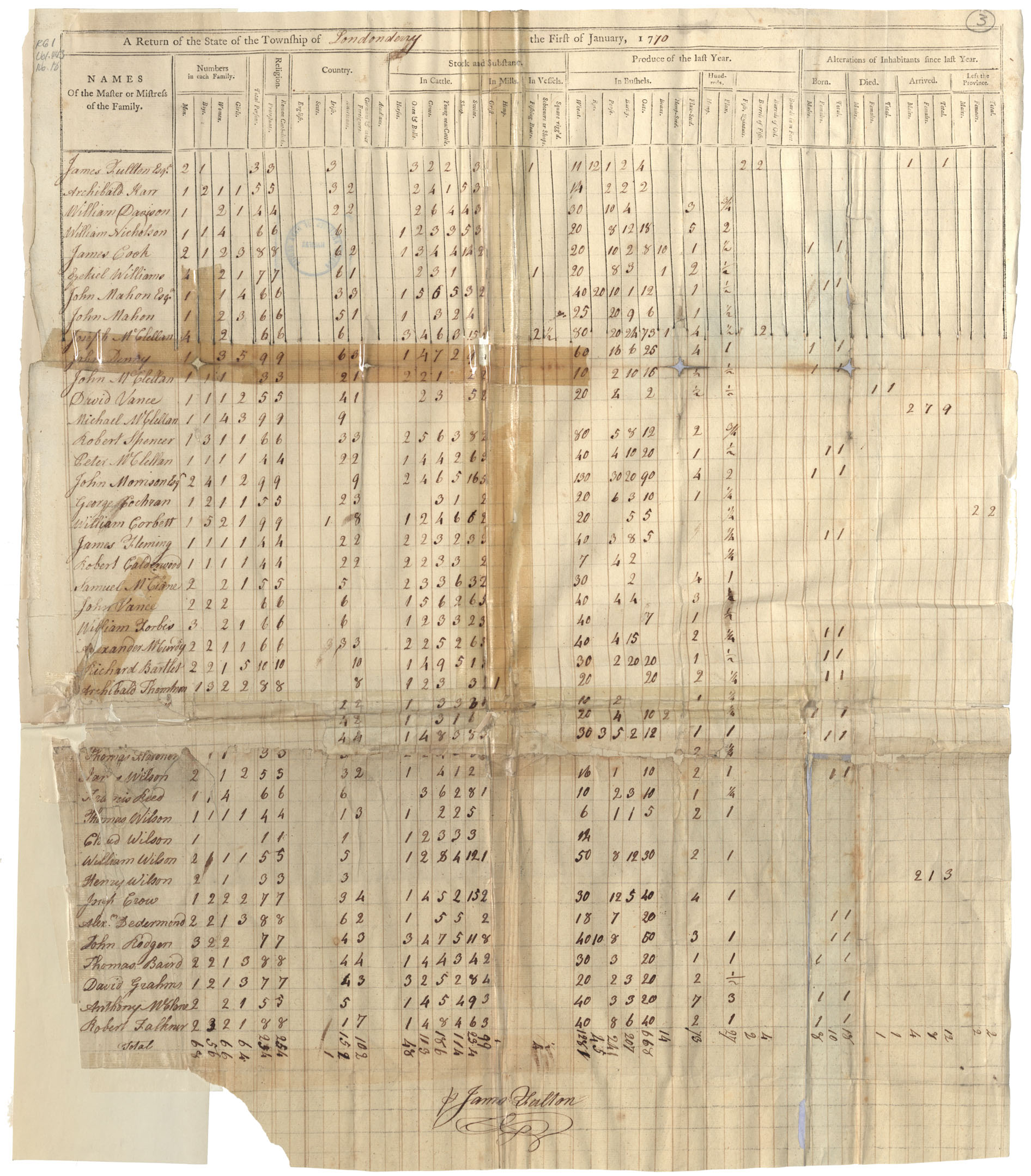The image depicts an aged, oxidized document, titled "The Return State of the Township of Londonderry" dating back to January 1st, 1710. The paper, delicate and heavily worn, has been reinforced with multiple strips of cellophane tape. One vertical tape runs from the top center to the middle, intersecting with a horizontal tape from the left side, and a diagonal tape section on the left forms a cross-like pattern. A torn piece remains at the bottom corner. This document resembles a census or immigration record, tracking family demographics. Columns on the left list names, with numerical entries to the right detailing family numbers, religious affiliations, country of origin, livestock, and more. Each column contains handwritten numbers in black ink. At the bottom center, a cursive signature, likely "James," authenticates the document. Additionally, a cursive inscription detailing sections and subentries runs throughout the paper.